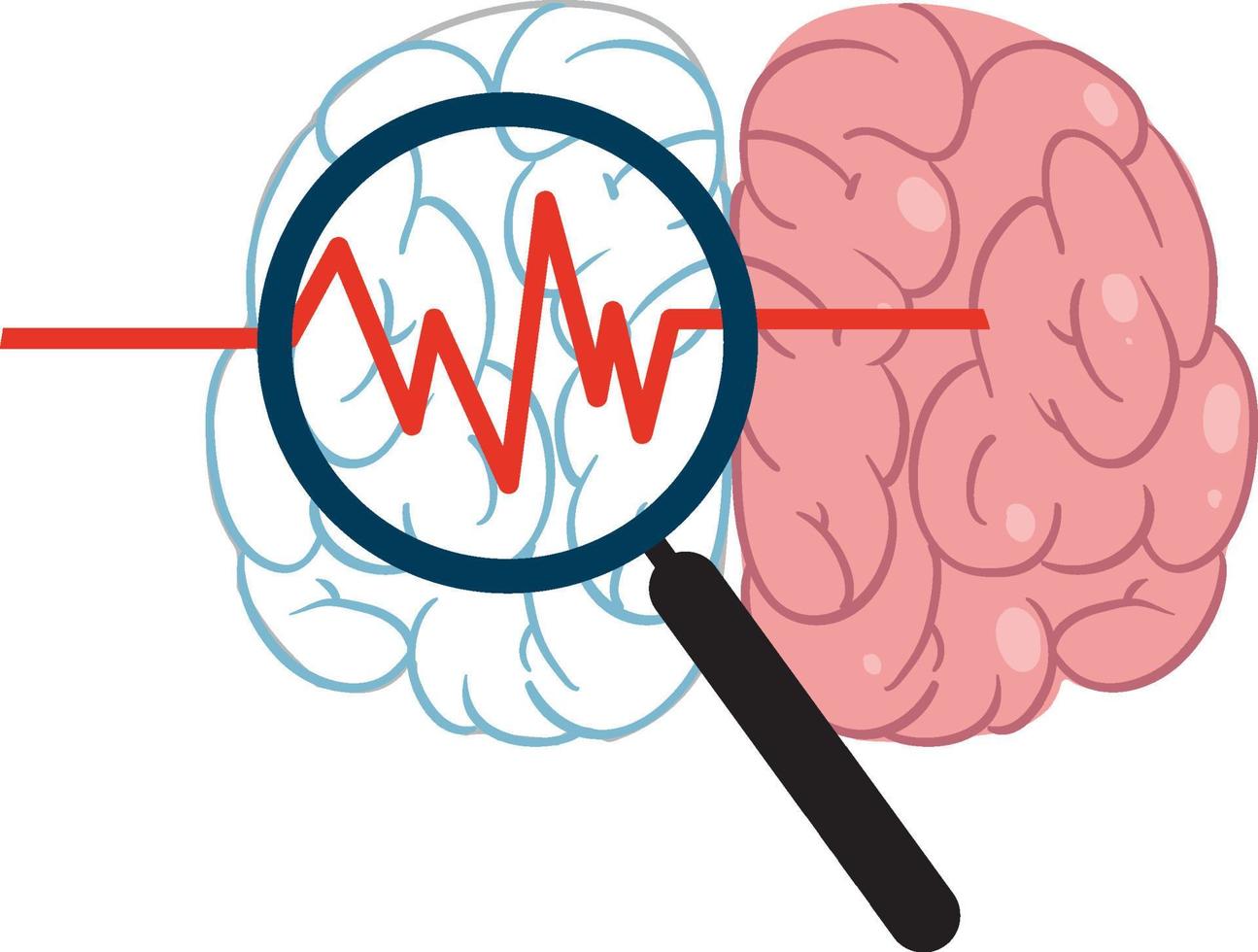The image depicts a stylized digital representation of two brain hemispheres. The left hemisphere is illustrated in a white to grey-blue palette, with various folds clearly outlined, giving it a more schematic or inactive appearance. The right hemisphere, by contrast, is vividly colored in shades of pink, resembling a healthy and active human brain. A magnifying glass, extending from the bottom right to the top left, hovers over the left hemisphere. Within the lens, a red line reminiscent of a heartbeat monitor shows jagged, dynamic activity, suggesting the inner workings or potential of the brain. This contrasts starkly with the flat line outside the magnifying glass, indicating a lack of activity. The overall composition, with its cartoonish yet detailed design, conveys a theme of examining brain functionality, possibly representing medical or scientific observation.